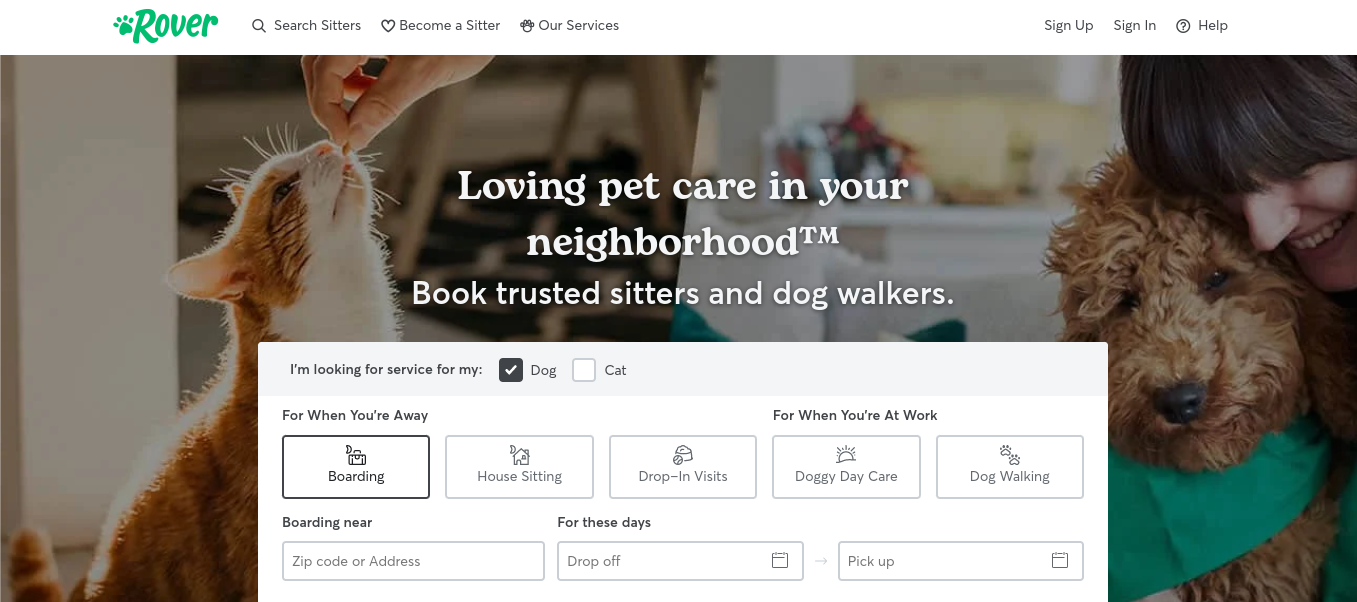This screenshot showcases the homepage of the Rover website, instantly recognizable by its logo in the top left corner: a green capital "R" with a paw print on the left side. The page features a split background banner image; the left half depicts a white and orange cat being fed a treat, while the right half shows a fluffy brown poodle being hugged by a smiling white woman.

Overlaying these images is text stating, "Loving pet care in your neighborhood™" followed by "Book trusted sitters and dog walkers." 

Below this text, a user-interactive form is present, helping visitors find pet care services. Part of this form is filled out, indicating that the user is looking for services for a dog. Below, service options are provided, including boarding, house sitting, drop-in visits, doggy daycare, and dog walking. Additional fields such as pick-up and drop-off details are also visible. The website is designed to be clear and user-friendly, emphasizing simplicity in navigation and functionality.